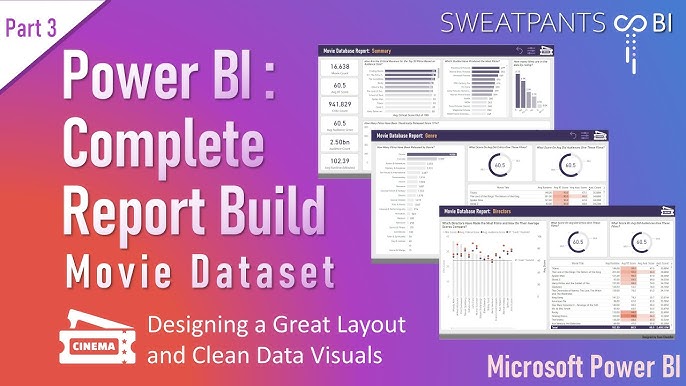This detailed advertisement for movie tickets has a vibrant gradient background transitioning from red on the left to pink, then to blue, and ending in purple on the right. In the top left corner, it prominently features the text "Part 3." Below this, large white letters spell out "Power BI," with subsequent lines reading "Complete Report Build" and "Movie Dataset." The bottom left corner showcases two cinema tickets, one partly obscured behind the other, with the visible ticket displaying an orange box labeled "Cinema" in white lettering. On the right side, there's text stating "Designing a Great Layout and Clean Data Visuals," accompanied by three screens displaying various indistinct diagrams and graphs. The top right corner features the text "Sweatpants BI" in white, while the bottom right corner also bears the white text "Microsoft Power BI."